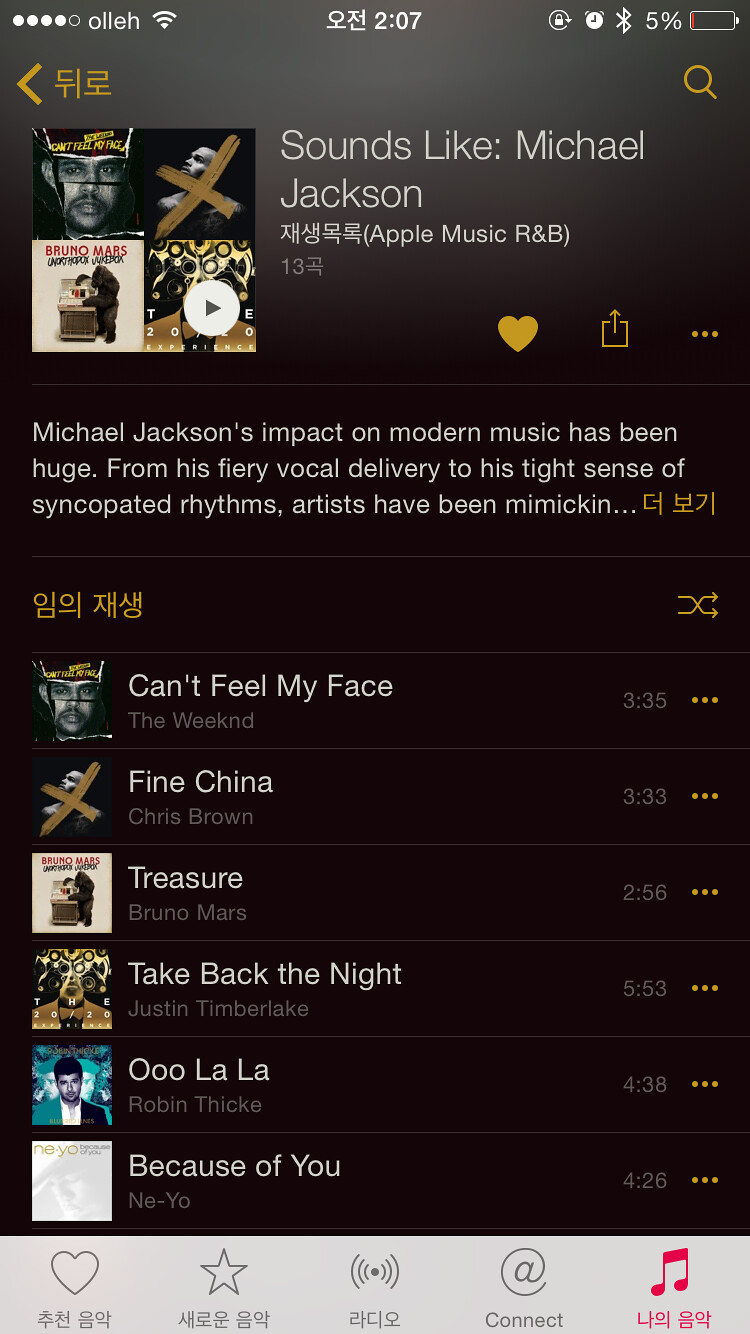The image depicts a tall, rectangular screenshot of an iPhone screen displaying the iTunes app. The background transitions from black to gray at the top. The phone is at 5% battery, indicated by the icon near the top-right corner, next to the time displayed as 2:07. In the top-left corner, an album cover is visible, composed of four smaller album covers. To the right of the album cover, in thin white font, it reads "Sounds like: Michael Jackson," followed by some Chinese or Korean symbols and the label "(Apple Music R&B)" in parentheses. Below this, a detailed paragraph begins with, "Michael Jackson's impact on modern music has been huge," and continues to discuss his influence, although part of the text is cut off.

The playlist seems to have songs that emulate Michael Jackson's style, featuring track titles and thumbnail images of the cover art. Notable songs listed are "Can't Feel My Face" by The Weeknd, "Fine China" by Chris Brown, "Treasure" by Bruno Mars, "Take Back the Night" by Justin Timberlake, "Ooh La La" by Robin Thicke, and "Because of You" by Ne-Yo. The display includes song durations and icons, with a column providing three dots either to the left or right of the song titles for additional options.